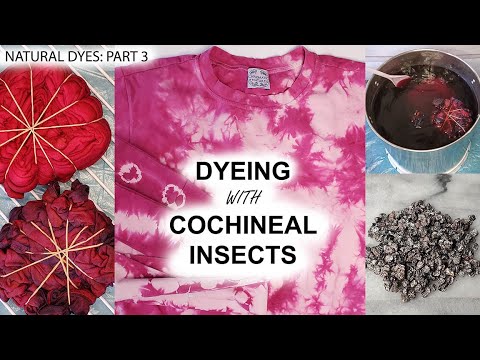This is an advertisement for a natural dye kit, depicted in a horizontally aligned rectangular picture with thick black borders on the top and bottom. The central feature of the image showcases a completed tie-dyed shirt in shades of red and pink, with a central faded white area overlaid with black text reading "Dyeing with Cochineal Insects" in all caps. 

To the left of the finished shirt, there are two other shirts bunched up and secured with rubber bands, dyed in varying shades of red and dark red, possibly with hints of black. Above this, in the upper left corner, the text "Natural Dyes: Part 3" is prominently displayed.

On the upper right side of the image, there is a silver galvanized bucket filled with a dark red liquid, with one of the tied-up shirts partially submerged and a plastic spoon in the liquid. Below this, on a gray and white marble countertop, is a collection of crushed cochineal insects in dried flake form, showcasing the raw material used to create the dye. The entire composition presents a vivid and detailed illustration of the natural dyeing process using cochineal insects.